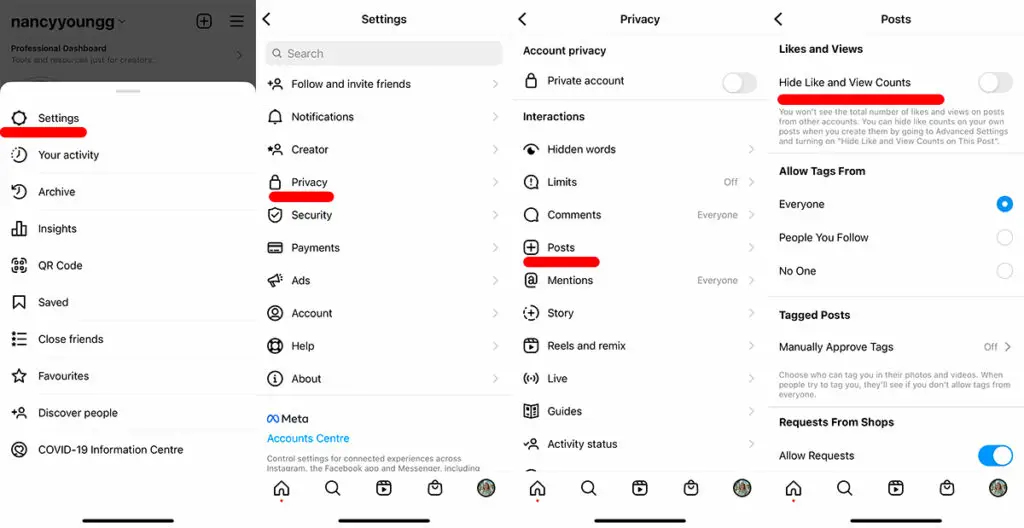The image is a composite of four sequential screenshots taken from a cell phone, arranged side by side, depicting a user navigating through the settings of an app.

1. The first screenshot on the far left shows the phone’s main settings page, with "Settings" displayed prominently at the top. Below this heading, the user’s account name "Nancy Young" (with two Gs) is partially greyed out, indicating that it is selected.

2. The second screenshot, positioned second from the left, displays the "Privacy" section of the settings menu. There is a noticeable red underline beneath the word "Privacy," suggesting that this is the current area being focused on.

3. The third screenshot, second from the right, delves deeper into the privacy settings. A bold red underline emphatically highlights the "Posts" section as the user navigates further into the options.

4. The final screenshot on the far right showcases the "Posts" settings page where the option "Hide like and view counts" is underlined in red. The feature's slider switch is clearly visible and shown in the off position, indicating that the user has the option to toggle it on or off.

This detailed sequence visually guides the viewer through the step-by-step process of configuring privacy settings within an app on a cell phone.